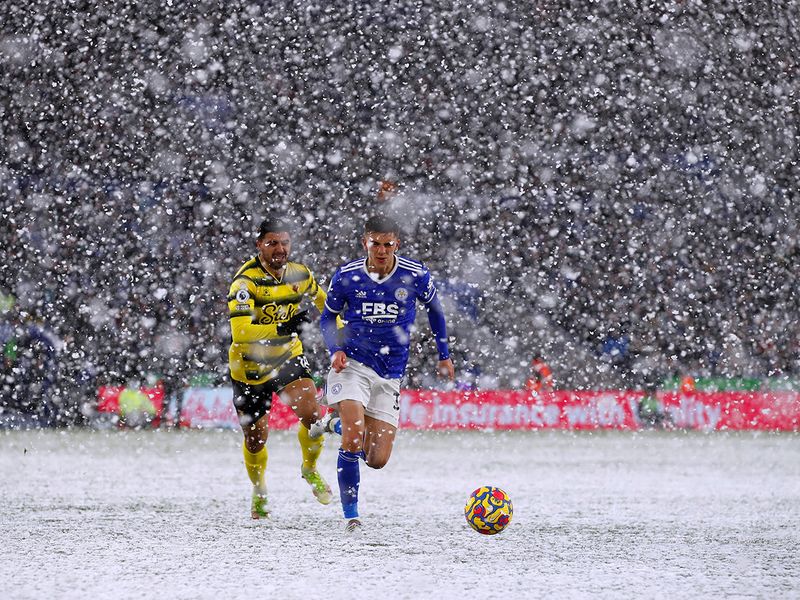In this dramatic image of a soccer match taking place amid a heavy snowstorm, two players are captured dynamically chasing after a vividly colored soccer ball with distinctive yellow, blue, and red accents. The player on the left dons a predominantly yellow and black striped jersey, obscured at the chest by his raised hands, with matching yellow socks pulled up to his knees and black shorts. His opponent wears a blue jersey featuring white lettering, with white striped shoulders, complemented by white shorts and blue socks. The intensity of their focus and movement towards the ball is palpable, despite the thick snowfall that heavily blankets the soccer field, obscuring even the grass beneath. The top of the photograph's background, shrouded in darkness due to the dense snowflakes falling relentlessly, makes it difficult to discern any spectators. A red sign with white lettering, barely legible through the blizzard conditions, can be faintly made out on the stadium wall. The snow appears to obscure the audience entirely, emphasizing the severity of the storm and the sheer determination of the players.